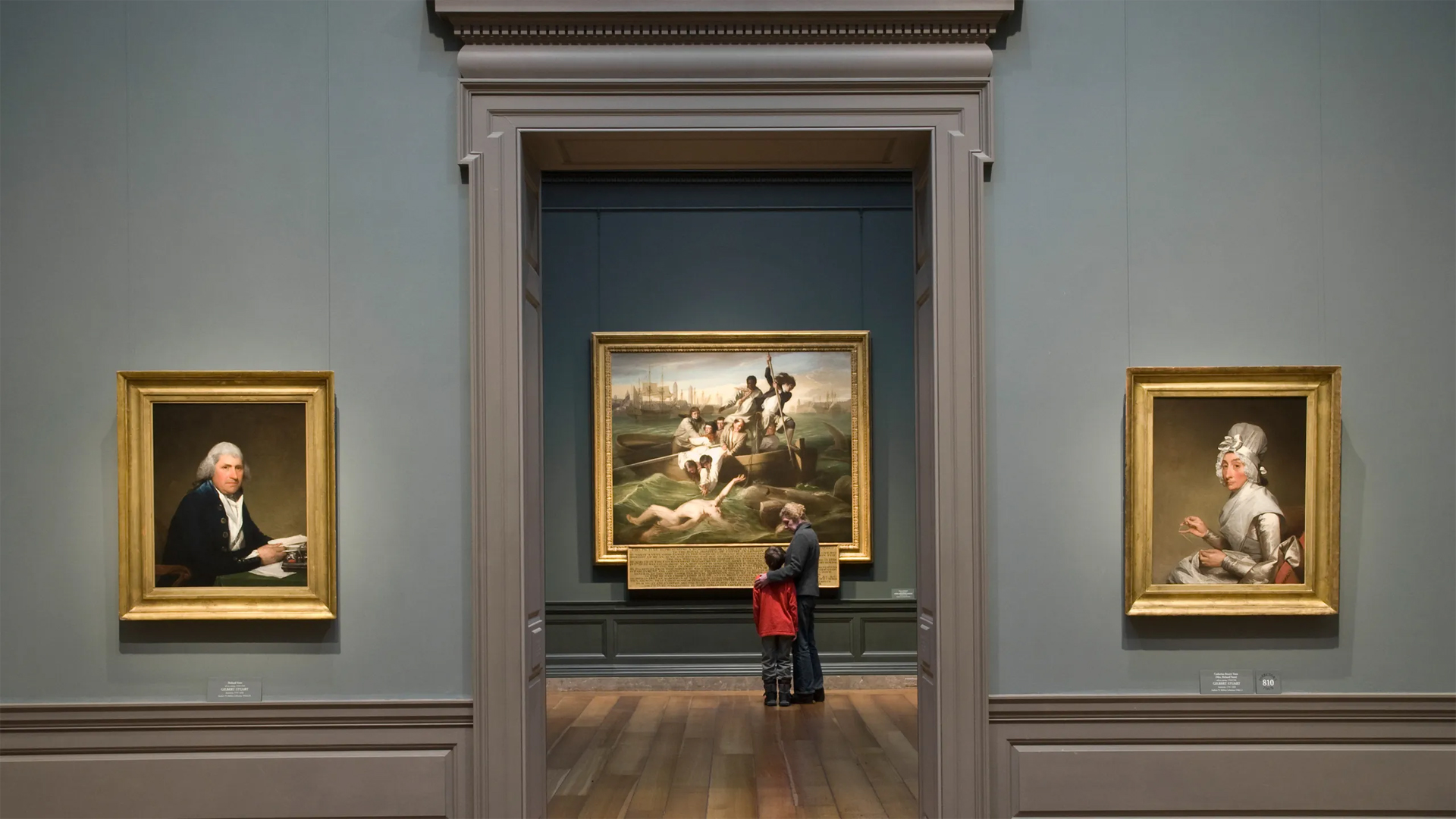In this photograph from an art gallery, we observe two rooms through an open doorway. In the foreground, the walls are depicted in light gray with darker gray paneling at the bottom. On the left side of this first room, framed in a gray frame, is a portrait of a man resembling Thomas Jefferson or George Washington, depicted in 1700s-style attire, wearing a black jacket and white shirt. On the right side, also framed in gray, is a Victorian-era woman with a wig, dressed in a grayish dress, reminiscent of the 1700s-1800s.

The doorway in the middle of these portraits leads the viewer's eye to a larger second room dominated by a vast Renaissance-style painting with a gold frame. This painting features a dramatic scene of men on a boat, with some falling into the water amid chaos, including one being stabbed. Standing in front of this gripping artwork in the second room are an elderly man and a young boy, presumably a grandfather and grandson. The boy, dressed in a red pullover, gazes at the powerful imagery as they stand against the backdrop of a grand golden-framed painting that takes up most of the gray-colored wall behind them.